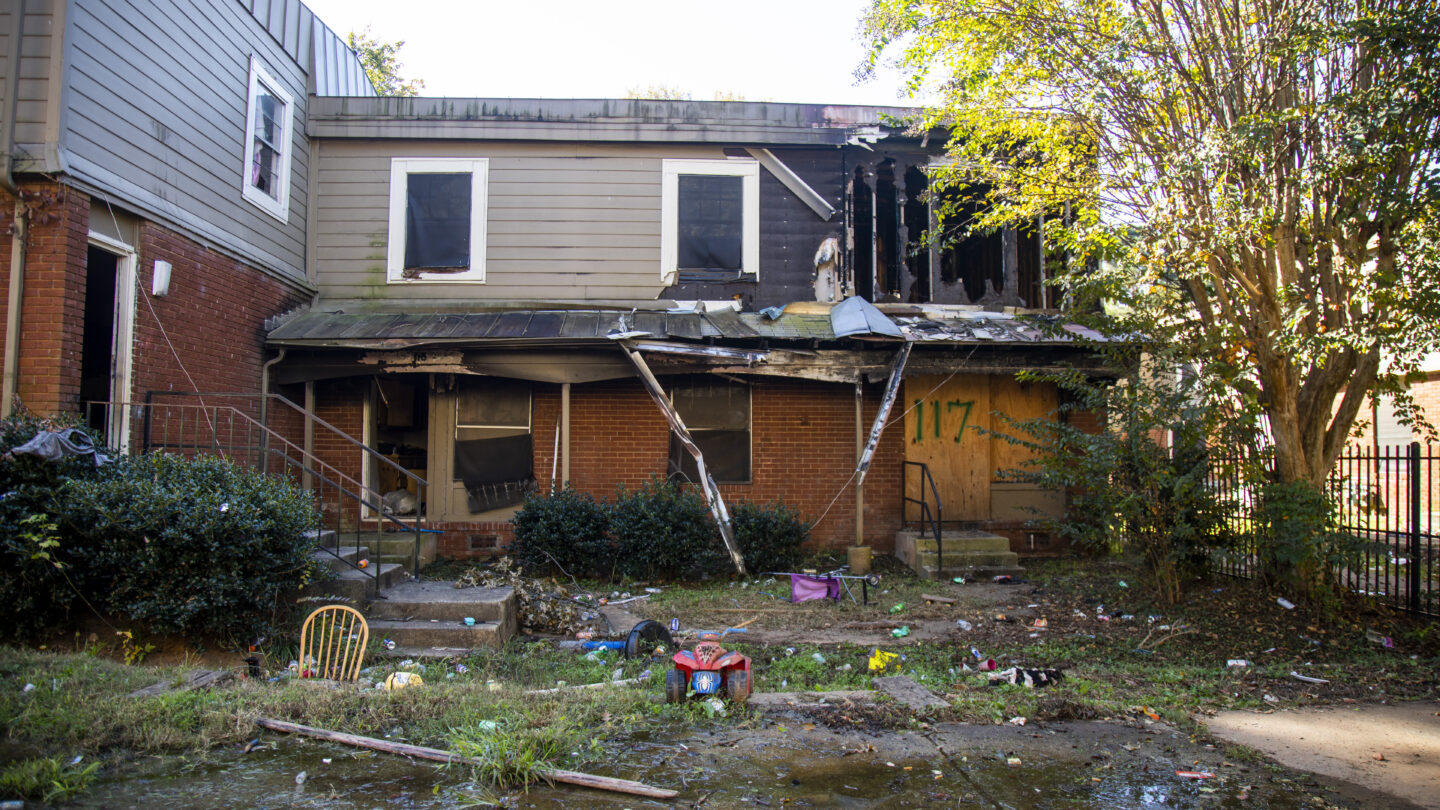This image depicts a severely run-down, two-story house that appears abandoned. The lower portion of the house features red brick, while the upper level has taupe-colored vinyl siding, some of which is missing, revealing black underlayment beneath. The right-hand side of the house displays noticeable fire damage. A doorway on the lower right is boarded up with plywood marked "117," and adjacent windows are either covered or broken with signs of burning. The front lawn, covered in dead grass and scattered trash, extends to the roof area. The backyard is cluttered with concrete slabs, children's toys, broken furniture, and standing water. A large tree stands to the right, next to a black iron fence that encloses the yard. The chaotic scene is further accentuated by the absence of a door in another entrance, replaced with overgrown bushes and stray trash, suggesting long-term neglect.